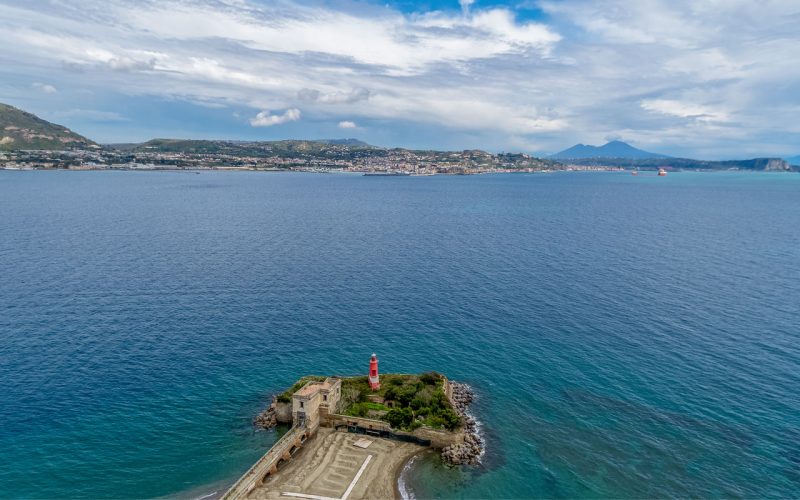This is an aerial photograph depicting a serene coastal scene dominated by a clear blue ocean. Centrally located in the foreground, a small peninsula juts out into the water. This peninsula features a prominent red and white lighthouse at its tip, edged by a rocky coastline and a triangular patch of green grass and trees. On the left side of the peninsula, a cement building and retaining wall are visible, while a sandy beach graces the right side. The horizon, positioned about two-thirds up the image, reveals a shallow, hilly peninsula stretching across the left side and transitioning into hilly, mountainous terrain towards the right. The distant landscape contributes to the depth and grandeur of the scene. White and light gray clouds predominantly blanket the sky, allowing occasional glimpses of blue. Adding to the coastal charm, small, indistinguishable boats can be seen far off on the horizon, enhancing the image's tranquil and expansive nature.